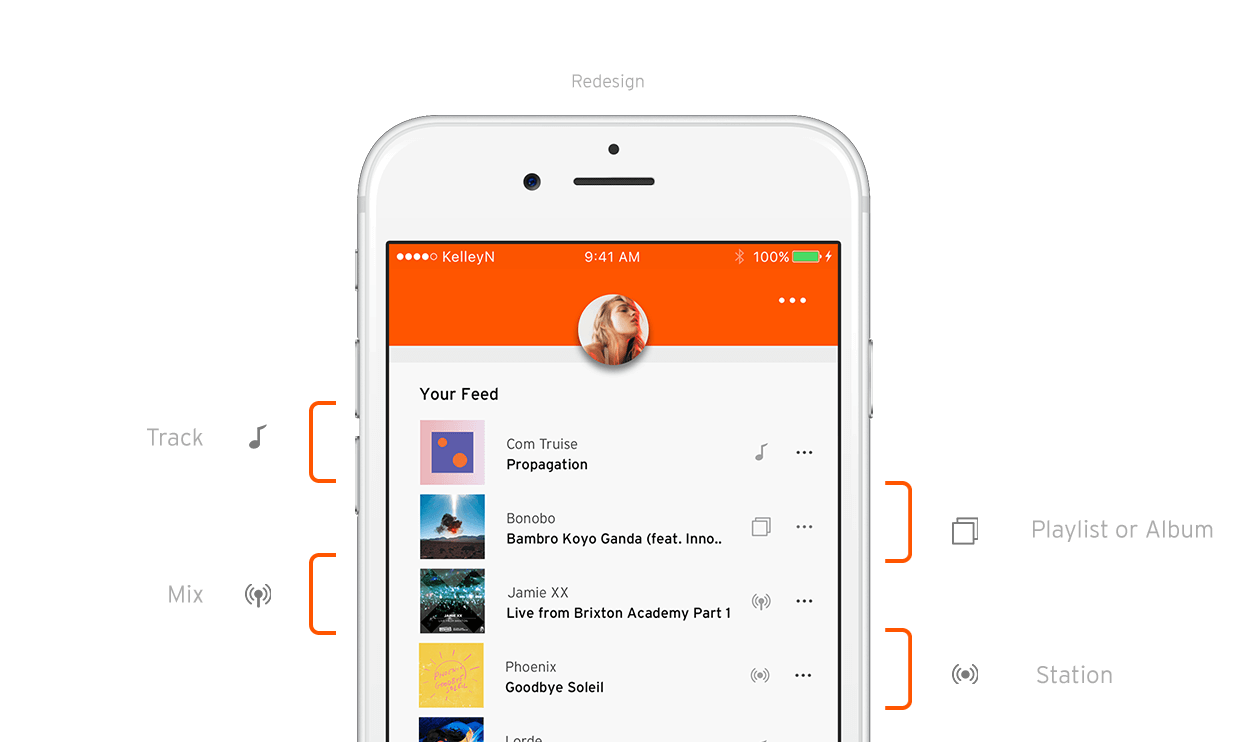**Detailed Caption:**

The image captures a white cell phone with a simulated display, demonstrating how content appears on its screen. The phone has distinctive black elements at the top center: a horizontal black line, a large black dot to the left of this line, and a smaller black dot above it.

The phone's screen showcases an interface, presumably of a music or media app, featuring a prominent bright dark orange banner at the top. On the left side of this banner, the signal strength and the carrier's name are displayed. The center of this banner shows the current time, while the right side includes the Bluetooth symbol, a green battery icon indicating 100% charge, and an ellipsis symbol (three dots) for more options.

Centered below the orange banner is a circular profile picture of a person with light brown hair looking upwards towards the top right corner. Beneath this profile picture, the feed section of the app is visible, displaying four completely visible thumbnails that resemble album covers, with a fifth thumbnail partially cut off at the bottom edge of the screen. Each thumbnail is accompanied by a light gray description and a bold line underneath it, presumably featuring additional information.

To the left side of the phone, outside the screen, an annotated orange staple points to two side buttons labeled "track" with a music note and "mix" next to a speaker or microphone icon emitting sound waves.

On the right margin of the screen, several options are listed with accompanying ellipsis symbols, including "copy" with three dots and a music note with three dots, among others.

Additionally, extending beyond the right edge of the phone, orange brackets are illustrated with labels: the top bracket features two stacked squares giving a 3D effect and is labeled "playlist" or "album", while the bottom bracket with a broadcast symbol is labeled "station".

This image was clearly created for instructional or training purposes, effectively demonstrating various on-screen and external phone elements for understanding app interface and phone functionality.